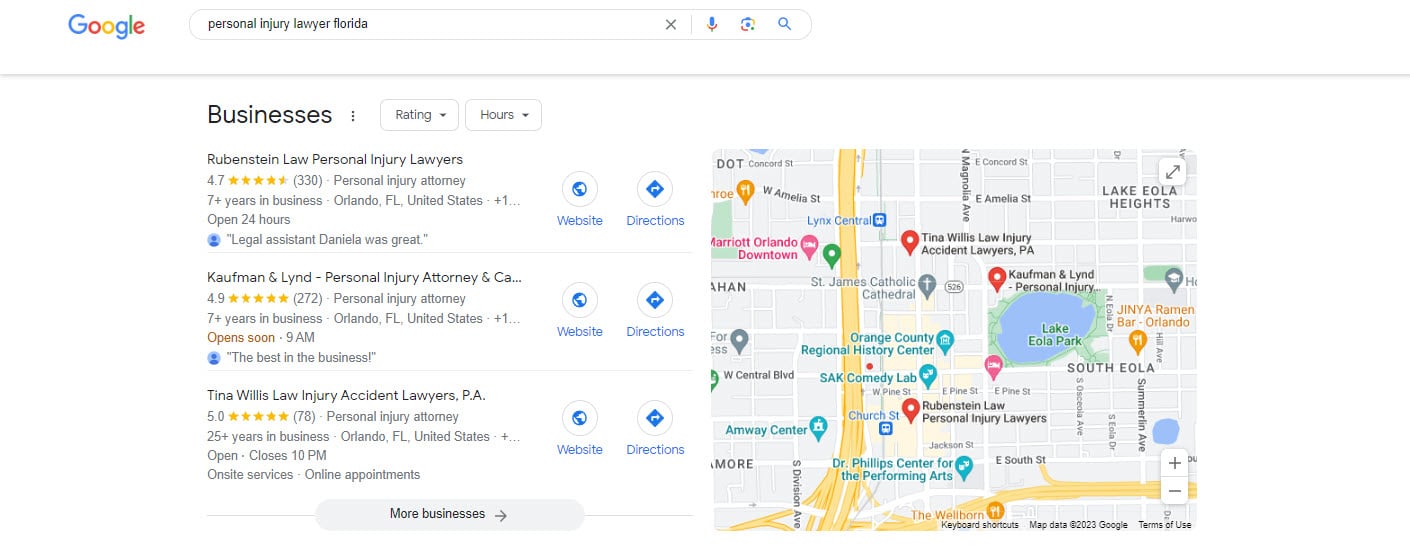The image showcases a Google search results page. In the top-left corner, the iconic Google logo is displayed in its signature blue, red, yellow, and green colors. To the right of the logo, a search bar is prominently placed, though the text inside is too small to decipher. Adjacent to the search bar are a microphone icon and a magnifying glass icon. Below these elements is a horizontal gray line spanning the width of the page.

Directly beneath this line, the word "Businesses" is written in black. To its right, there are two small, blurry text boxes. Proceeding downward, the page lists three search results. Each result features a pair of buttons—a "Website" button on the left and a "Directions" button on the right. Below these options is a larger gray button labeled "More," although the full text is not entirely legible.

To the right of the search results, the image includes a map highlighting two intersecting interstate highways and a nearby water body, either a pond or a small lake. Several red location pins are also visible on the map, indicating specific points of interest.